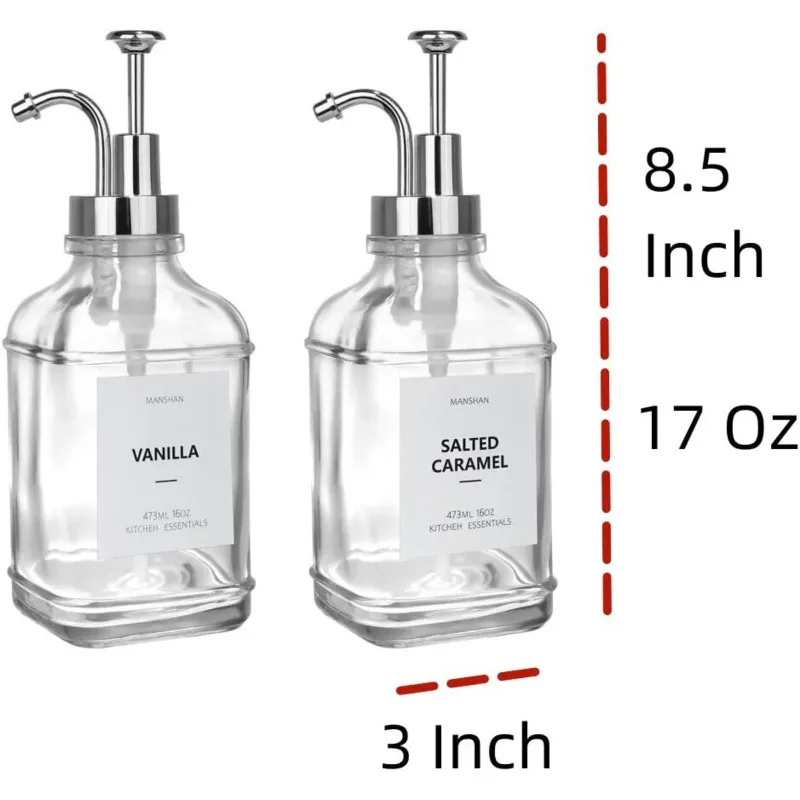This photograph depicts two elegant glass syrup dispensers placed side by side against a white background, commonly seen in coffee shops. Both dispensers feature a square base that tapers into a round top, each crowned with a chrome metal pump. These pumps consist of a circular disc, a rod, and a bent faucet-shaped spout from which the syrup is dispensed. Each clear glass jar has a white label with black text; the one on the left reads "Vanilla" and the one on the right reads "Salted Caramel." To the right side of the image, red dotted lines indicate dimensions: each dispenser stands 8.5 inches tall, is 3 inches wide across the base, and holds 17 ounces of liquid. The overall impression is of sophisticated and functional design, well-suited for stylish beverage preparation.